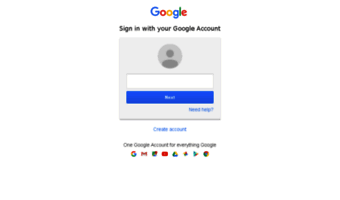A very small image depicts a Google sign-in page with "Google" prominently displayed at the top in its colorful font. Below this, there is a generic profile icon resembling the silhouette of a man's head and upper torso. The page includes a field where users can enter their username and a blue "Next" button to proceed to the password entry. Additional options on the page include "Need help?" and "Create account" links. At the bottom, a message reads "One Google account for everything," highlighting the interconnectedness of Google's services such as Gmail, Maps, YouTube, and Drive. The overall background of the page is a clean white or light gray, maintaining Google's signature simple and user-friendly interface.